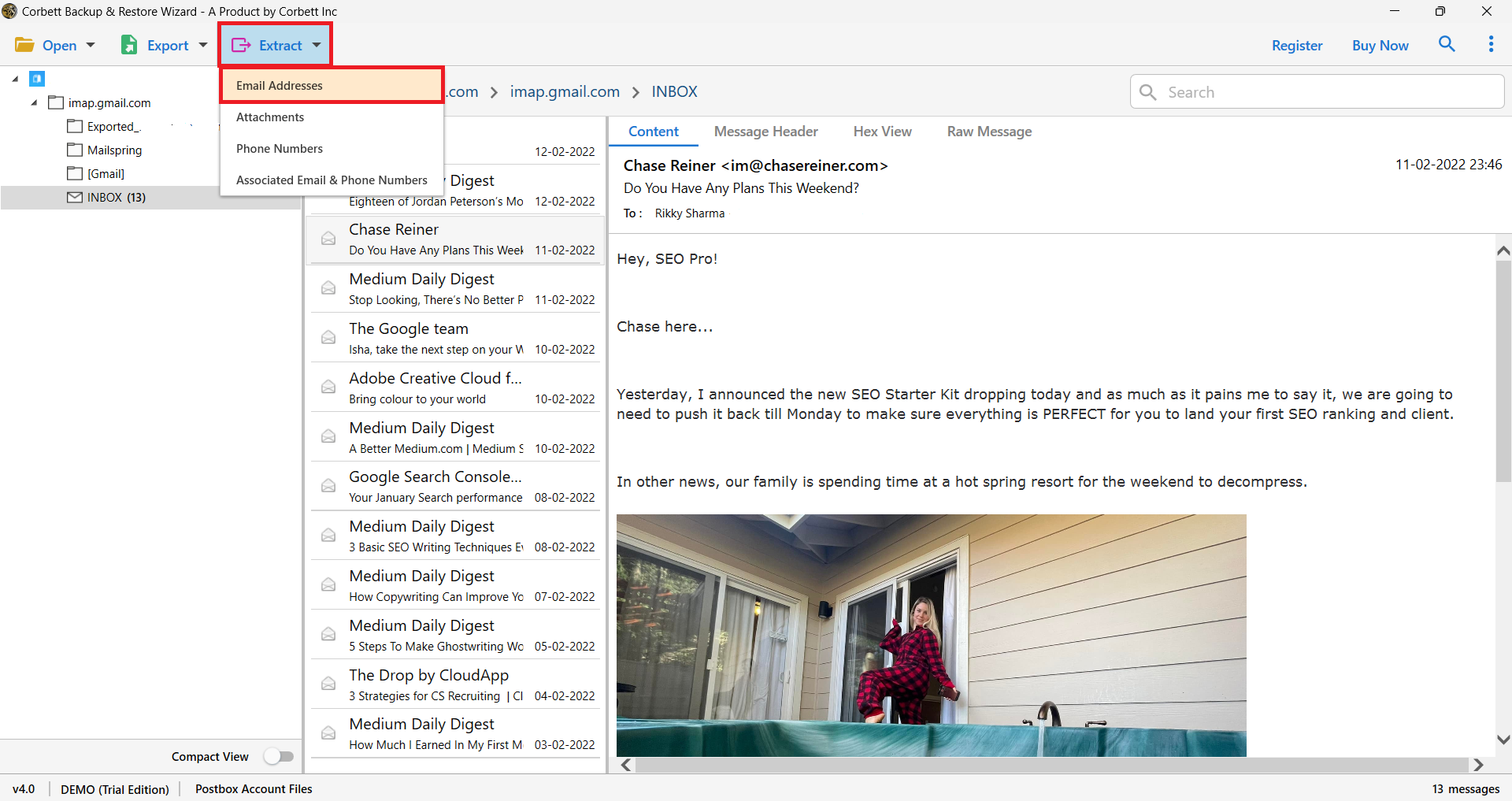The image is a screenshot from a computer showing the interface of the Corbett Backup and Restore Wizard, a product by Corbett Incorporated. Prominently displayed at the top of the screen is the software's title. In the center, within a red rectangular outline, is the "Extract" button, marked by a blue label next to an icon resembling a paper with a right-pointing arrow.

Below the "Extract" button is a drop-down menu that includes options such as "Email Addresses," "Attachments," "Phone Numbers," and "Associated Email and Phone Numbers." The option "Email Addresses" is selected, highlighted in a pale orange color with a red border outlining the selection box.

On the left side of the screen, there is a list of emails. The selected email is from Chase Renner, addressed to "Hey SEO Pro." The email begins with, "Chase here. Yesterday, I announced the new SEO starter kit dropping today and as much as it pains me to say it, we are going to need to push it back till Monday to make sure everything is perfect for you to land your first SEO ranking and client."

Additionally, the email contains an image of a person wearing black and red flannel, positioned next to a woman by a hot tub. The overall scene captures the user interface of the software effectively while providing a detailed view of the selected email content.